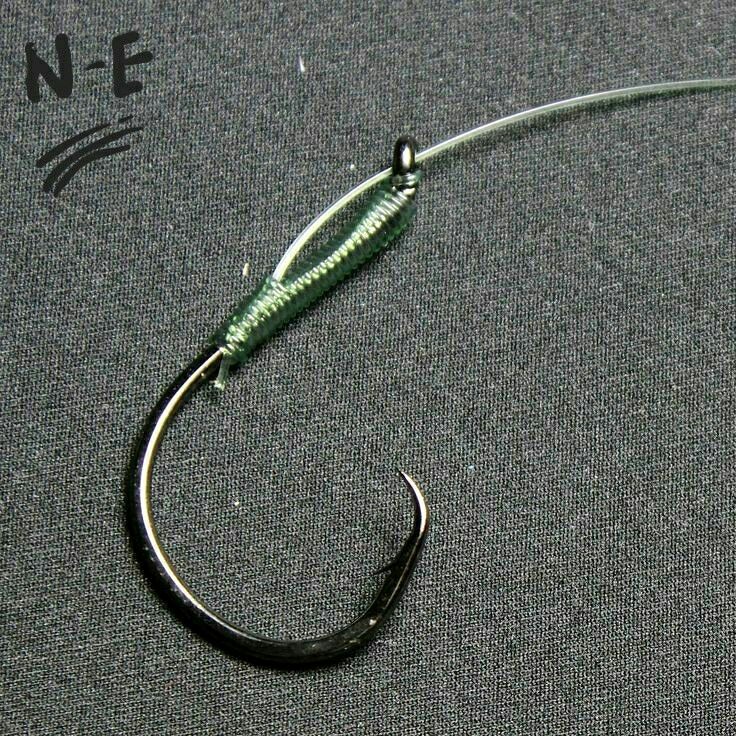The image is a large square photograph featuring a textured gray fabric background, providing a heathered appearance. In the upper left corner, "N-E" is handwritten in black marker, with three diagonal, curved lines beneath it. Dominating the center of the image is a metal fishing hook. The hook starts from the upper right corner, curves through the middle to the lower left, and then arcs back up to the center. This detailed fishing hook has a light green area near its top, where an eye for threading a fishing line can be seen, alongside a silver-tipped black point at the bottom. Despite its ornamental elements, the hook itself lacks the additional features typical of a fishing lure.